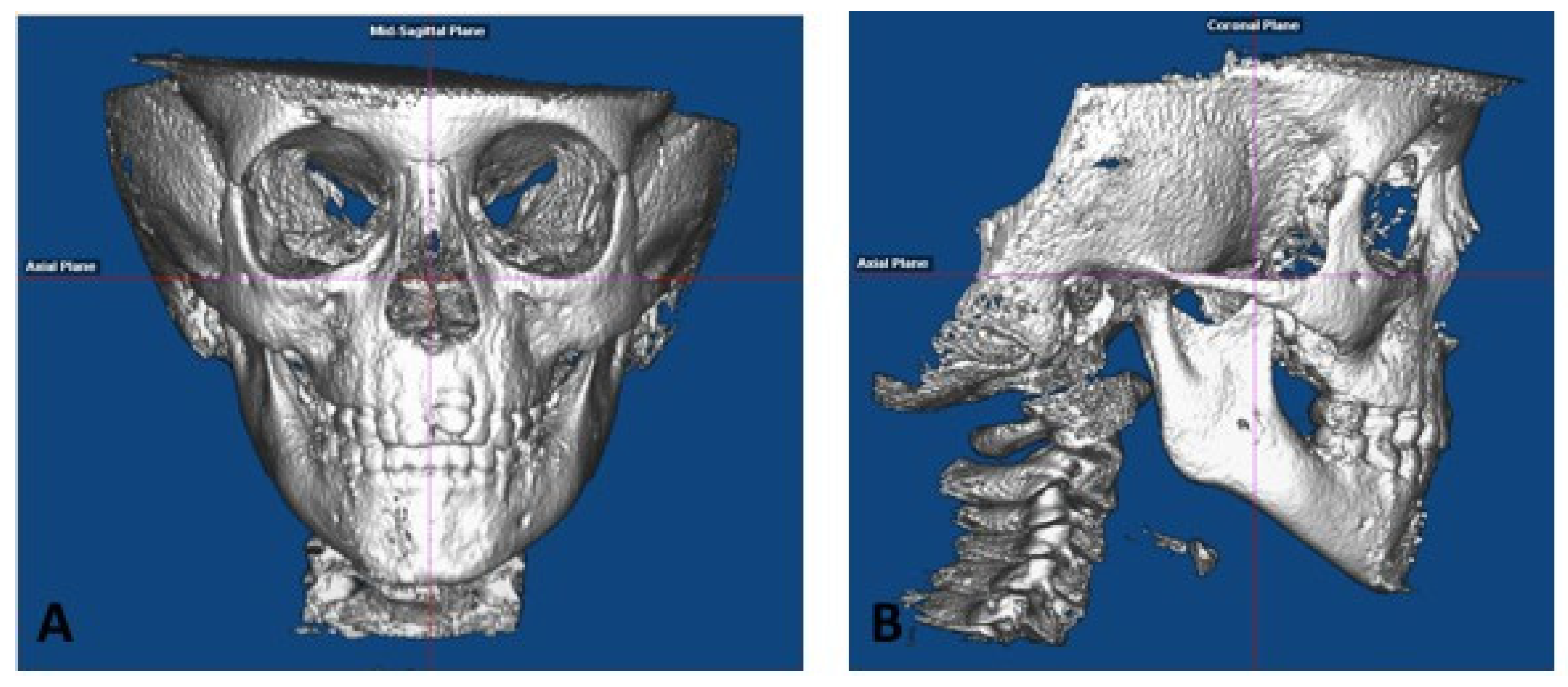The image comprises two 3D-rendered, silver-colored, partial skulls set against a deep blue background. On the left, labeled 'A', the frontal view is displayed, showing an anatomical depiction of a skull from the eyes down to the neck, with prominent eye sockets, full teeth in a closed mouth, and a visible section of the spine. On the right, labeled 'B', a side profile of the same skull reveals a pointy jawline and detailed neck contours. Both images have intersecting red lines marking reference points vertically and horizontally, along with some unreadable medical annotations. The top portion of the skulls, from the eyes upward, is missing, giving an eerie appearance, and emphasizing the anatomical structure from the eyes to the spinal connection.